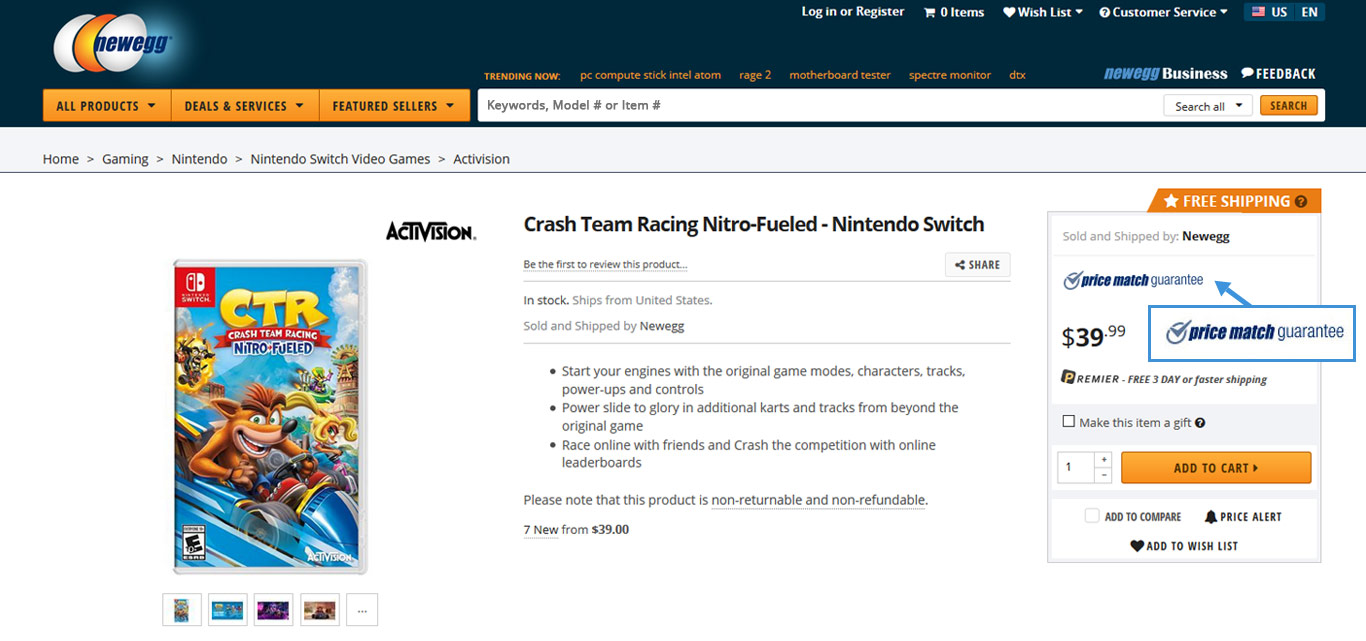Here is a cleaned-up and detailed caption for the image:

---

The Newegg website features a dark blue background with a prominent logo in the top-left corner. The logo comprises a series of eggs in white, yellow, and orange hues, with the "Newegg" text in blue superimposed on the eggs. 

At the top-right corner of the page, there are several user interface elements including options to log in or register, a cart displaying zero items, a wish list, customer service links, and language settings set to U.S. English. 

Below the Newegg logo, there are navigational buttons featuring pull-down menus labeled "All Products," "Deals," and "Seller Features." 

Centrally positioned is a white search bar with the prompt "Keywords, Model Number, or Item Number." Directly below "Trending Now" is highlighted in orange font with popular items such as "PC," "Compute Stick," "Intel Atom," "Rage 2," "Motherboard Tester," and "Spectrum Monitor DTX" listed underneath. Next to the search bar on the right, there's an "Orange Search" button and a note about Newegg Business Feedback.

The highlighted item for sale is "Crash Team Racing Nitro-Fueled for Nintendo Switch," which is currently in stock and available for shipment within the United States. The product is sold and shipped by Newegg. A blurb beneath the product announcement reads: "Start your engines with the original game's mods, characters, tracks, power-ups, and controls. Power slide."

---

This caption captures the layout and specific details of the Newegg webpage described.